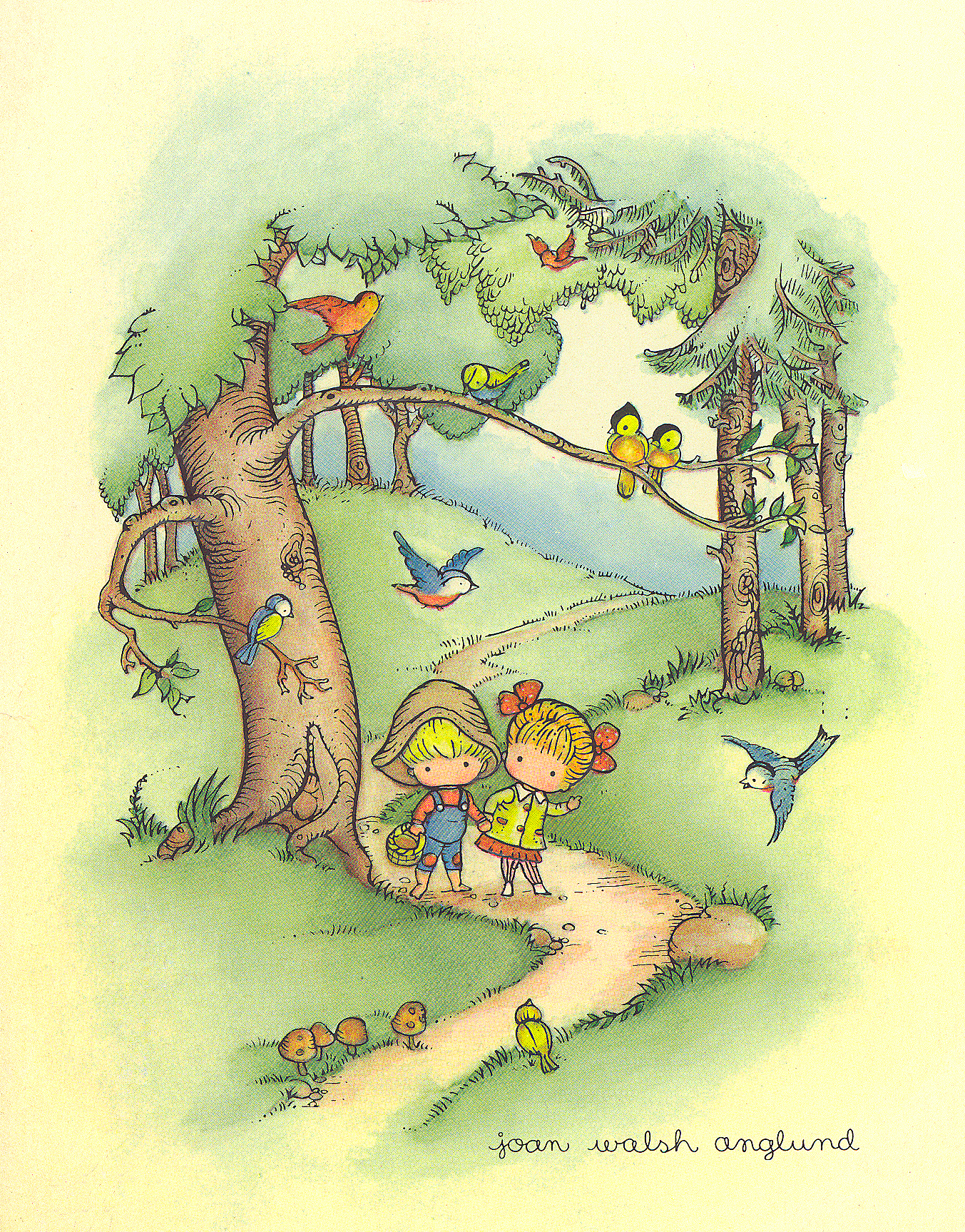The image is a digitally created cartoon portrait, with a signature at the bottom right that reads "Joan Walsh Anglund" in cursive. It depicts a serene woodland scene, vibrant with various birds and nature details. At the center, a young boy and girl are holding hands as they walk down a dirt path. The boy is wearing a hat and a blue and red outfit, while the girl is dressed in a red skirt and a yellow vest. The surroundings are lush with green grass hills and multiple trees with brown trunks and leafy green canopies. 

Birds are plentiful in this scene: a green and blue bird, a blue and yellow bird perching on a lower branch with its blue back and yellow chest, a red bird higher up on the same tree, alongside three small yellow birds near the branch's end. Additionally, there are red birds dotting the grove, including one flying in the sky. The presence of brown mushrooms adds to the woodland feel. On the right-hand side, there are three tall trees, likely evergreens, with visible trunks and lower portions of their green foliage completing this picturesque scene.